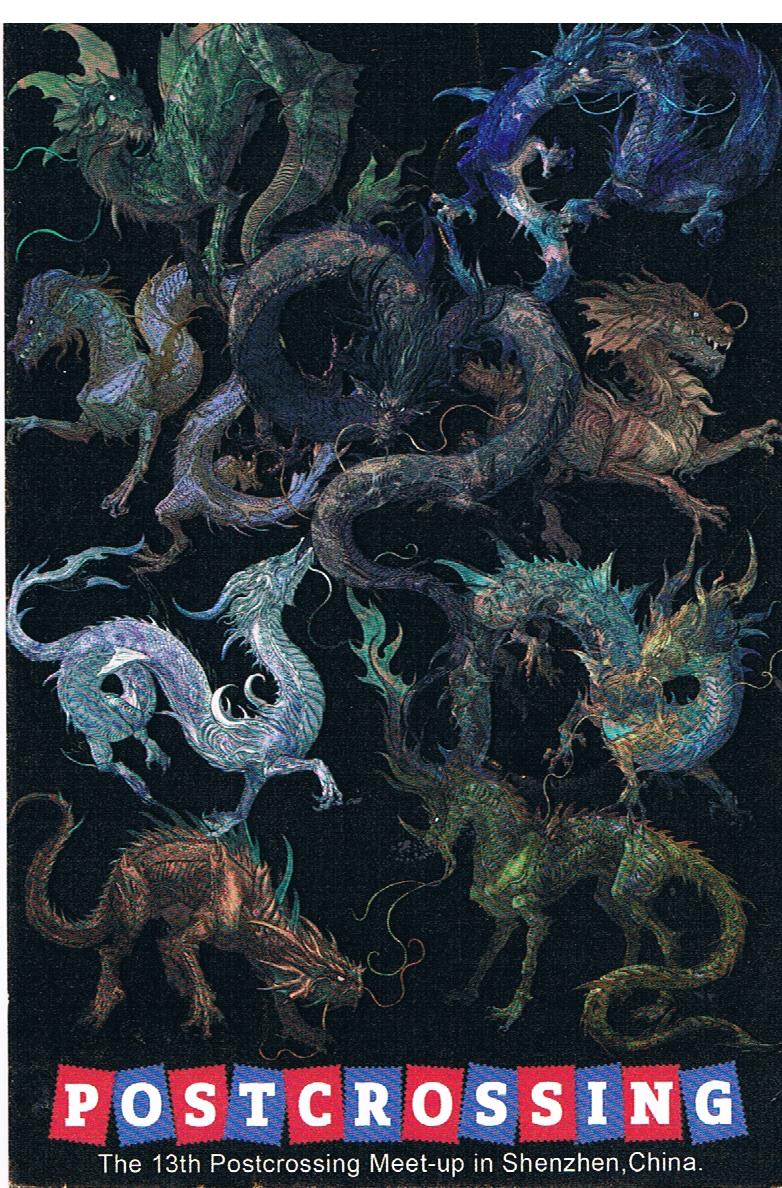This poster commemorates the 13th Post-crossing meetup in Shenzhen, China. Dominated by intricate drawings of various Chinese dragon figures, the poster features a dazzling array of dragons in a multitude of colors including brown, green, light blue, dark blue, and gold, all against a stark black background. The dragons exhibit a wide range of styles, from opulent, ornamental designs to more menacing, monster-like creatures. Some dragons are serpent-like, coiled and flying, while others are depicted with four legs, resembling mythical Chinese dragon horses. In the upper right corner, a symbol of a creature hangs down, and to the upper left, a dark green coiled lizard figure stands out. The bottom part of the poster showcases the word "post-crossing" in white letters, each within a red or blue square, reminiscent of vintage movie theater signs. Below this, in plain white text, the event details are clearly stated: "the 13th Post-crossing Meetup in Shenzhen, China."